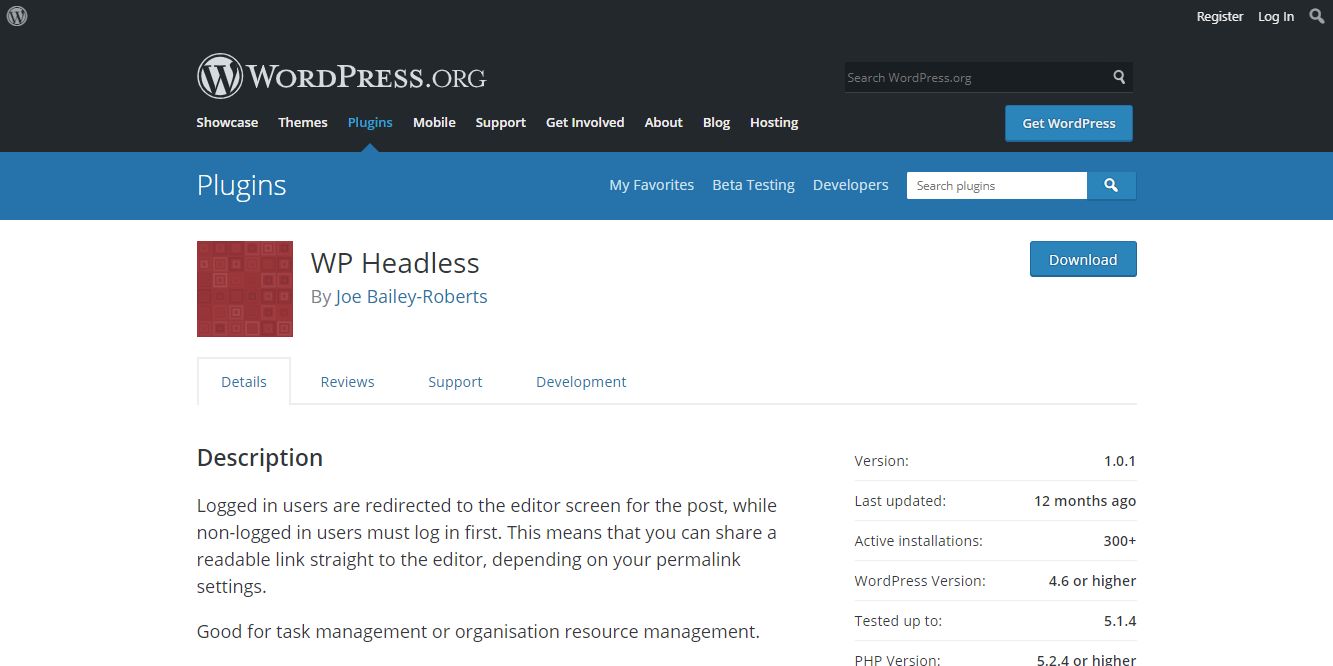This is a detailed screenshot of the website wordpress.org. At the top, there's a prominent black bar featuring the WordPress logo, a white circle with a black "W" at its center, followed by the text "wordpress.org" in white. Adjacent to this, there's a black search bar containing a search icon.

Below this header, there's an extensive navigation menu comprising several options: Showcase, Themes, Plugins (which is highlighted), Mobile, Support, Get Involved, About, Blog, and Hosting. Towards the right end of the nav bar, there is a prominent blue rectangular button labeled "Get WordPress."

Directly beneath the navigation menu, there's a thin horizontal bar with the title "Plugins." To the right of this title, there are categories including "My Favorites," "Beta Testing," and "Developers," along with another search bar specific to this section.

The main content area of the screen has a white background. Centered at the top, the title "WP Headless" is displayed. To the left of this title, there's a small maroon square icon with multiple smaller squares inside it. Underneath the title, the author is credited as "Joe Bailey Roberts," and to the right, there's a blue "Download" bar.

Below this header, there are four tabs labeled "Details," "Reviews," "Support," and "Development," followed by a description section. The description notes: "Logged in users are redirected to the editor screen for the post, while non-logged in users must log in first. This means that you can share a readable link straight to the editor depending on your permalink settings. Good for task management or organization resource management." Further down, there are additional details including the version number "1.0.1," the last update timestamp of "12 months ago," active installations, and other pertinent plugin information.